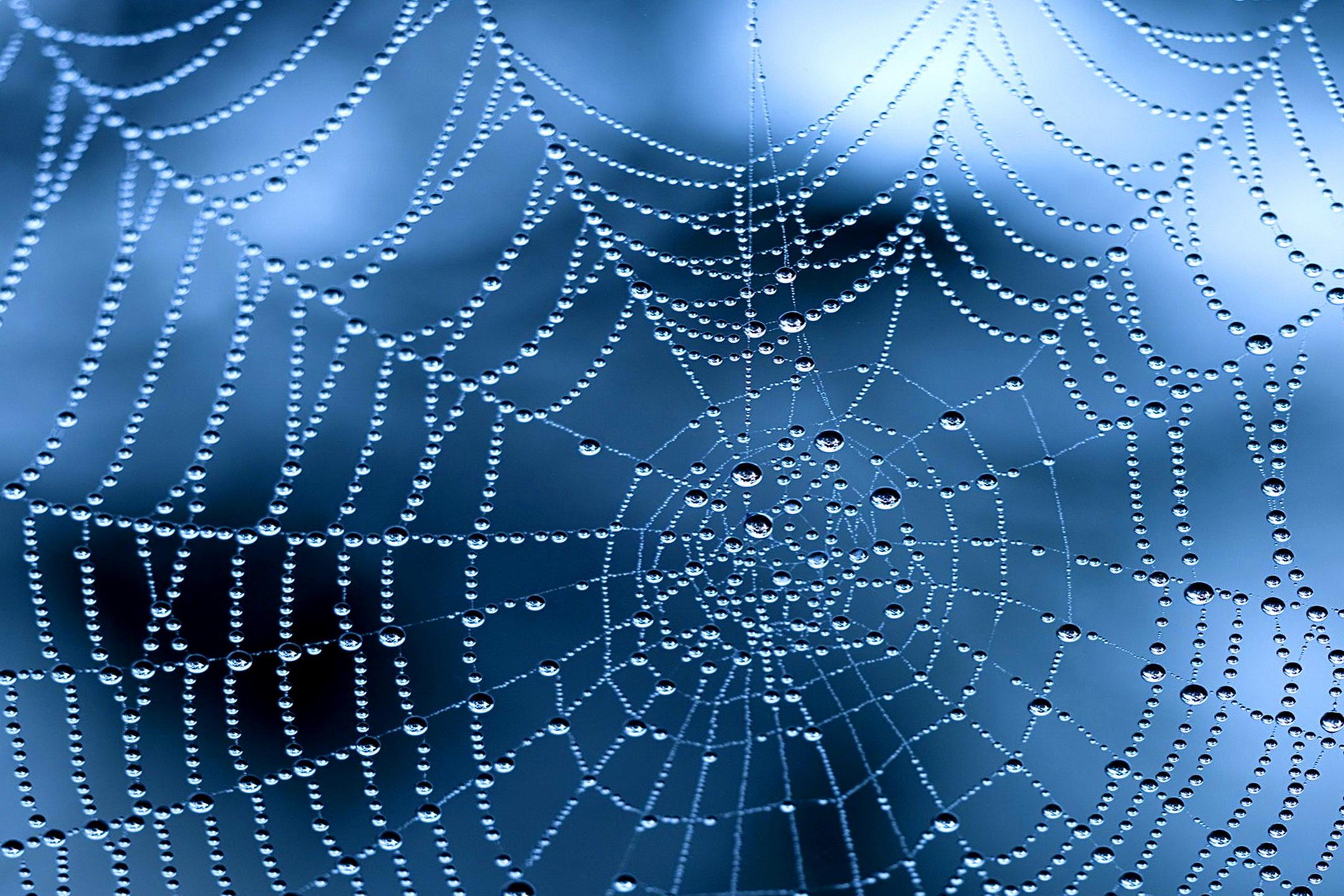This image showcases a detailed spider web intricately designed with what appears to be small, bead-like water droplets. The web, predominantly white, features an intricate pattern of interconnected lines forming a round shape, with the center being the thickest and most densely packed area. The middle of the web is positioned just right of center and slightly lower than the midpoint of the image. The web’s structure consists of outward-branching lines formed by slightly larger beads, which are then connected by smaller beads, creating a complex, delicate network. The background, visible through the web, is a blend of blurry blue, white, and dark blue patches, adding a soft, diffused contrast to the striking web.